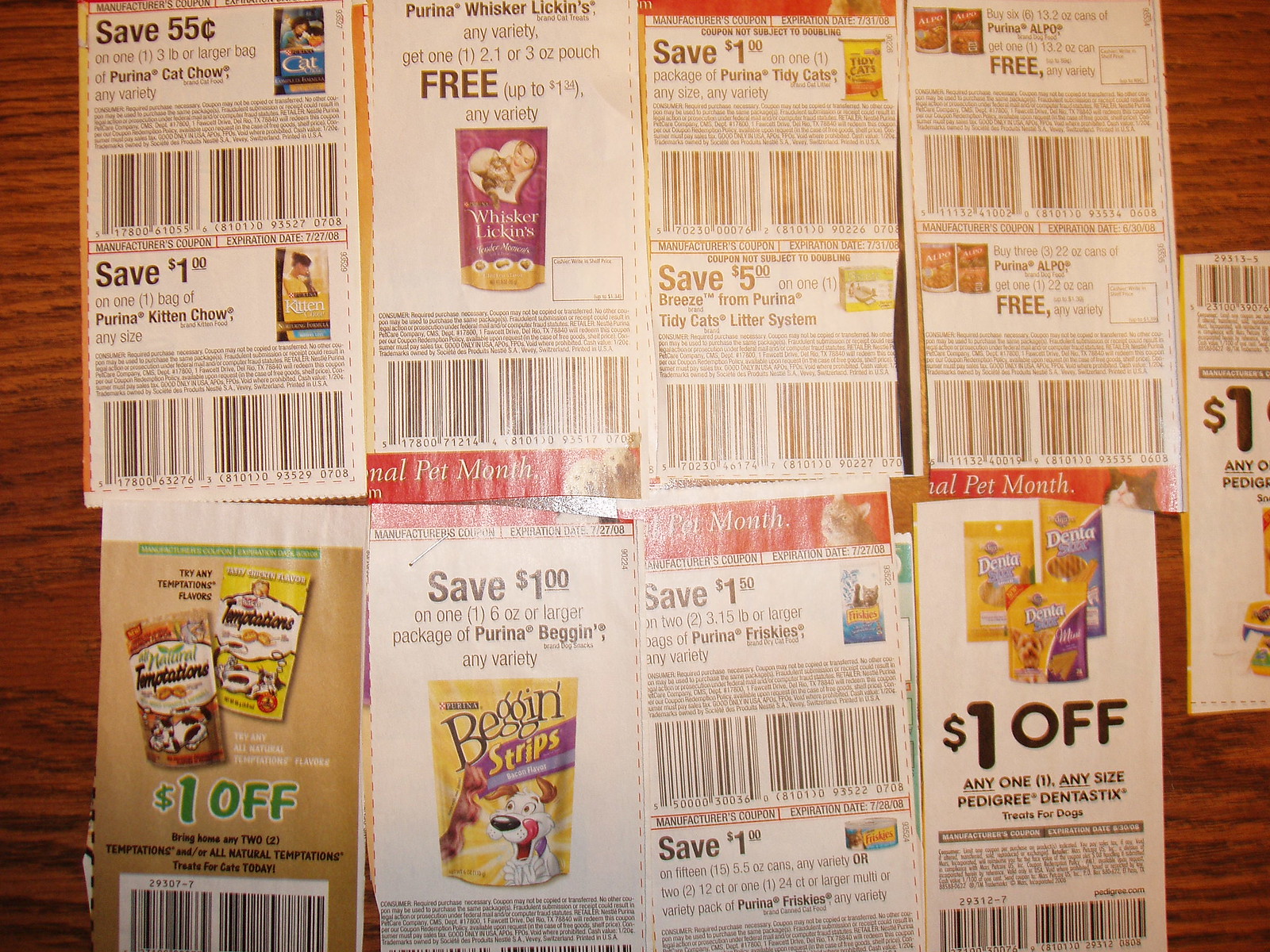This image features nine clipped coupons meticulously arranged atop a medium-brown, wood-grained tabletop. The coupons are placed in two neat rows of four, with the ninth coupon positioned to the right between the two rows. Each coupon is dedicated to pet-related products, including well-known brands such as Purina and Pedigree. Specifically, one can identify coupons for Purina Kitten Chow, Purina Alpo, Tidy Cats Litter, Purina Friskies, Pedigree Dental Sticks, Beggin' Strips, and Temptations. The details on the eighth coupon are unclear, but it's consistent with the pet theme. While most coupons offer dollar-off discounts, there is one standout in the upper row with a generous $5 off. The entire ensemble is carefully displayed, emphasizing the variety and potential savings for pet owners.